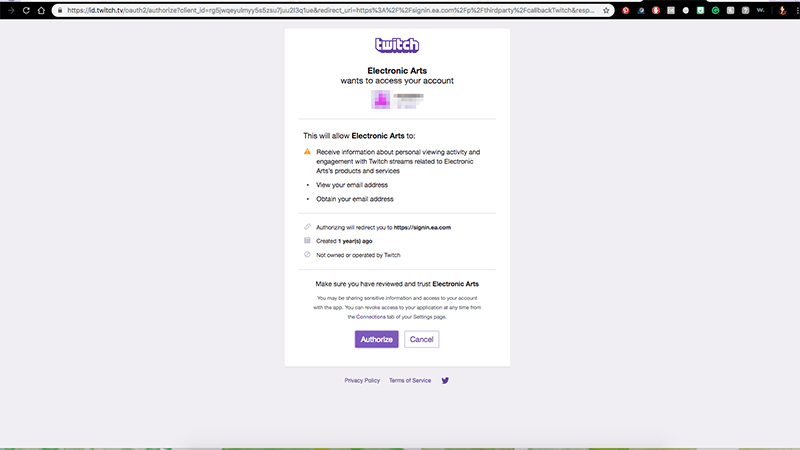The image depicts a screenshot of an account authorization page for Twitch and Electronic Arts (EA). The interface has a gray background, with a URL displayed at the top. At the top right corner, there is a set of icons on a black background. In the main section of the screen, there is a prominent white box framed by the larger gray background. 

The white box contains a request message from Electronic Arts (EA), asking for access to the user’s Twitch account. The message explains that granting access will allow EA to receive information about the user’s personal viewing activity and engagement with Twitch streams related to EA products and services. Additionally, EA will obtain the user’s email address. 

A note indicates that authorizing this access will redirect the user to the URL https://signin.ea.com. The information also states that this URL was created a year ago and is not owned or operated by Twitch. Users are advised to review and trust Electronic Arts before proceeding.

Below this message, there are two buttons: a purple button with "Authorize" written in white letters, and a white button with "Cancel" written in purple letters. At the bottom of the white box, there are links to the Privacy Policy and Terms of Service, alongside a blue-purple colored bird icon representing Twitter.